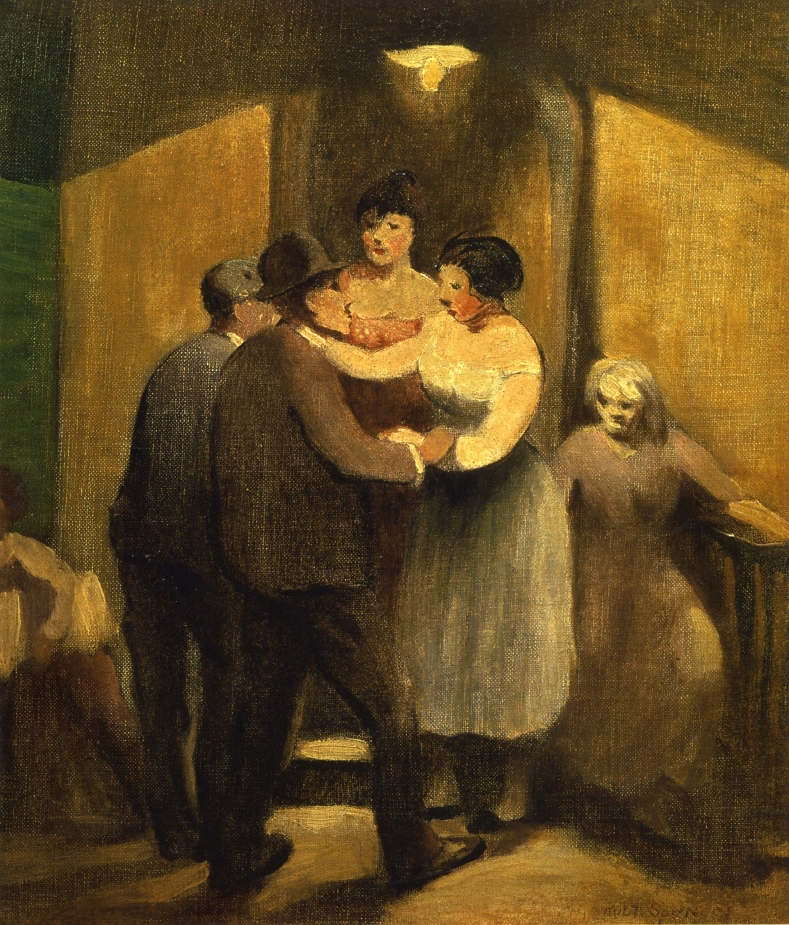The painting portrays a night scene in front of a building with a yellow wooden background, possibly a pub, illuminated by a streetlight attached to the structure. Six individuals of Caucasian, European descent are depicted with rough, textured brushstrokes that obscure detailed facial features. 

In the center, a woman in a white long-sleeve shirt and a long blue skirt clasps the shoulder of a man beside her. This man, dressed in a black dress jacket, white collared shirt, black pants, black shoes, and a black bowler hat, reciprocates by clasping her right forearm. Behind them stands another woman in a pink dress, seemingly observing the man in the bowler hat. 

Towards the doorway, which is beneath a glowing yellow light, two women engage with two men. One woman, attired in white and red dresses with her hair pulled back, is positioned in the doorway, suggesting interaction under the arch. Close to her, a woman in an orange dress sits atop a step, slightly elevated from the rest, hinting at a casual gathering ambiance. 

Next, a man in a brown suit and derby hat places his right hand on the left hand of the woman in white, while she rests her right hand on his left shoulder. Near them, another man in a black or possibly blue suit, wearing a similar hat, observes the scene. 

To the far right stands an elderly woman in a long tan dress with white hair, leaning on a railing. She appears to be observing the interactions around her, her gaze directed to the left, towards the group. The scene's cohesive palette of tan, neutral white, and gray tones unify the ensemble, delivering a detailed narrative of a seemingly intimate moment captured in rustic hues.